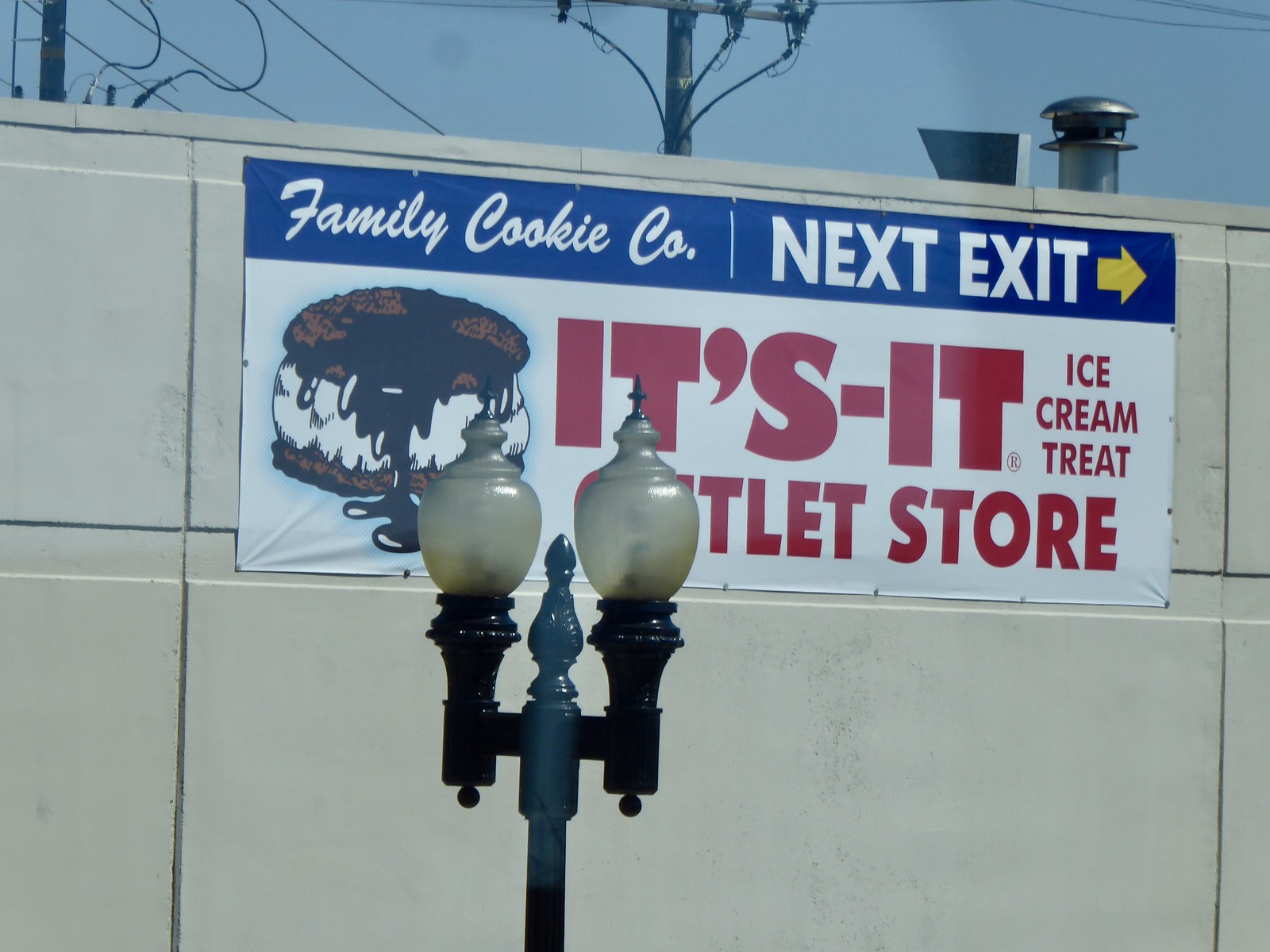In the image, we see the side facade of a building prominently featuring a large, eye-catching sign near its upper edge. Atop the building, a smokestack rises into the sky alongside a network of power lines. In the foreground, a streetlight with two lamps adds to the urban ambiance of the scene. The most striking element of the photograph is the vibrant sign for the "Family Cookie Company," displayed in elegant cursive lettering. The sign includes an inviting message, "Next Exit," accompanied by a bright yellow arrow directing potential customers. Featured prominently on the sign is a tempting image of an ice cream sandwich crafted from cookies, with delectable chocolate dripping down its sides. Below the image, bold red letters announce "It's It Outlet Store," followed by the phrase "Ice Cream Treat" to entice dessert lovers. The overall composition of the image combines elements of urban infrastructure with a vivid advertisement that captures the viewer's attention.